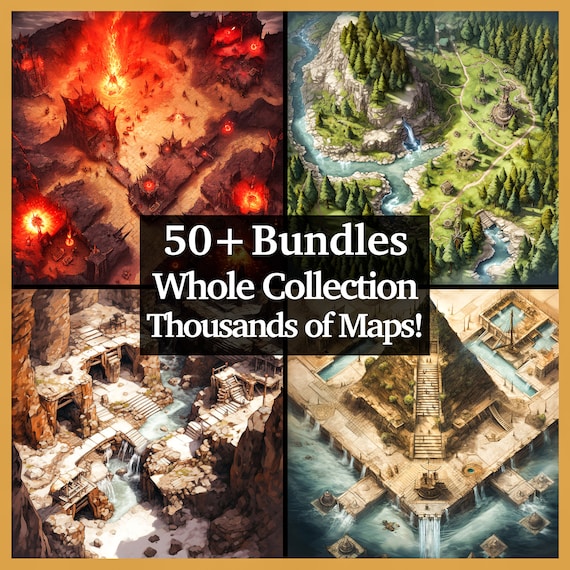The image features a gold-bordered square divided into four distinct sections, each showcasing a unique scene. In the center of the square, a black triangle background displays the text "50+ BUNDLES" in white font, accompanied by "WHOLE COLLECTION" beneath, followed by "THOUSANDS OF MAPS!" in capital letters with an exclamation point.

In the upper left corner, there is a depiction of a fiery lava explosion within a volcano, with flames and eruptions vividly illustrated. The upper right corner presents a serene landscape of a green valley, characterized by a meandering river flowing through lush trees and grass, leading to a central waterfall.

The bottom left corner reveals ancient rock ruins carved into the side of a mountain, devoid of any inhabitants, evoking a sense of historical mystery. The bottom right corner showcases a pyramid-like temple structure set on a tan base, surrounded by water. The pyramid features central stairs ascending towards the top, with tiny figures suggesting people climbing the stairs.